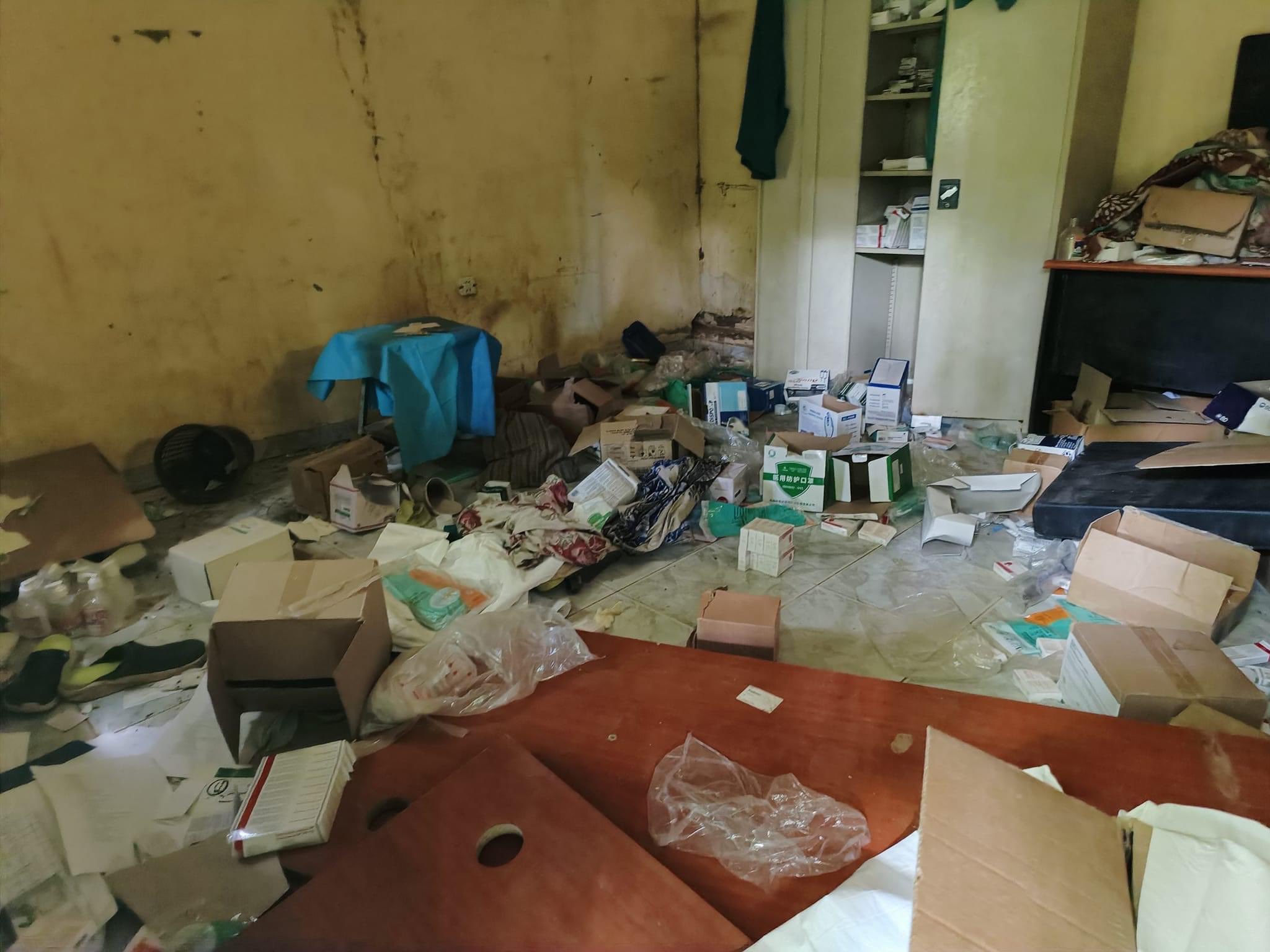This photograph depicts an extremely cluttered and disorganized room. In the background on the left, a worn and water-damaged beige wall is evident, marked by a large brown stain down the center and a grey stain near the bottom. On the right side of the image, a similar wall is partially obscured by a large, slightly olive green metal cabinet. One door of the cabinet is ajar, revealing shelves filled with boxes, while the other door remains closed. 

Adjacent to the cabinet on the right side is a wooden desk with a brown top and a black base. The desk is heaped with an assortment of cardboard and fabric. Spanning the remainder of the floor are large marble-style tiles arranged in squares, strewn with a chaotic array of bags, boxes, shoes, bottles, and various other items. 

A stool or chair appears on the left side of the image, draped with a blue piece of fabric. In the foreground, two reddish-brown pieces of wood are placed at angles to each other near the bottom left corner. Each piece of wood features a hole roughly the size of a drinking glass. Overlaying these wooden pieces is a clear piece of plastic. Additionally, a rectangular piece of brown cardboard rests on top of white paper or plastic bags in the bottom right corner of the image.